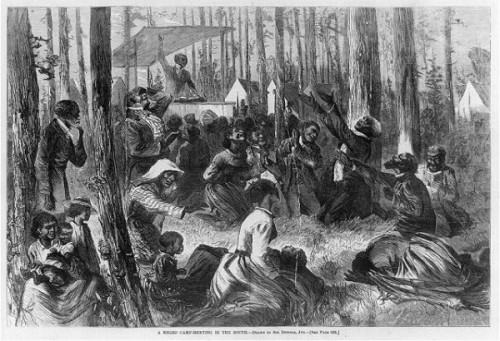This black-and-white drawing vividly captures a tense and emotional scene set in a dense forest. At its core, the artwork portrays a group of people, attired in Victorian-era clothing, including women with feathered hats and men in greatcoats. Central to the image are two women who are tied down on their knees, surrounded by other women, some of whom have children. These children display various emotional reactions, from burying their faces in their hands to gazing upwards with outstretched arms, as if pleading for divine intervention.

The periphery of the scene includes individuals leaning against trees, reinforcing the sense of a communal gathering amidst nature. Dominating the background is a man standing behind a podium-like structure, possibly a preacher, delivering a fervent sermon. His right arm is raised high towards the sky, and a black object rests on a white table in front of him. 

The forest’s trunks are starkly visible, but the branches and leaves fade into the indistinct backdrop. Additionally, there are glimpses of a small village with white-walled houses, one of which features a triangular rooftop, hinting at a distant community life. A solitary wagon suggests recent travel or preparation for a journey, adding to the narrative depth.

The entire scene exudes a sense of historical tension, perhaps indicative of a sermon or gathering during slavery times. Text too small to read is present at the bottom of the drawing, and the overall composition is both emotionally charged and rich in period detail.